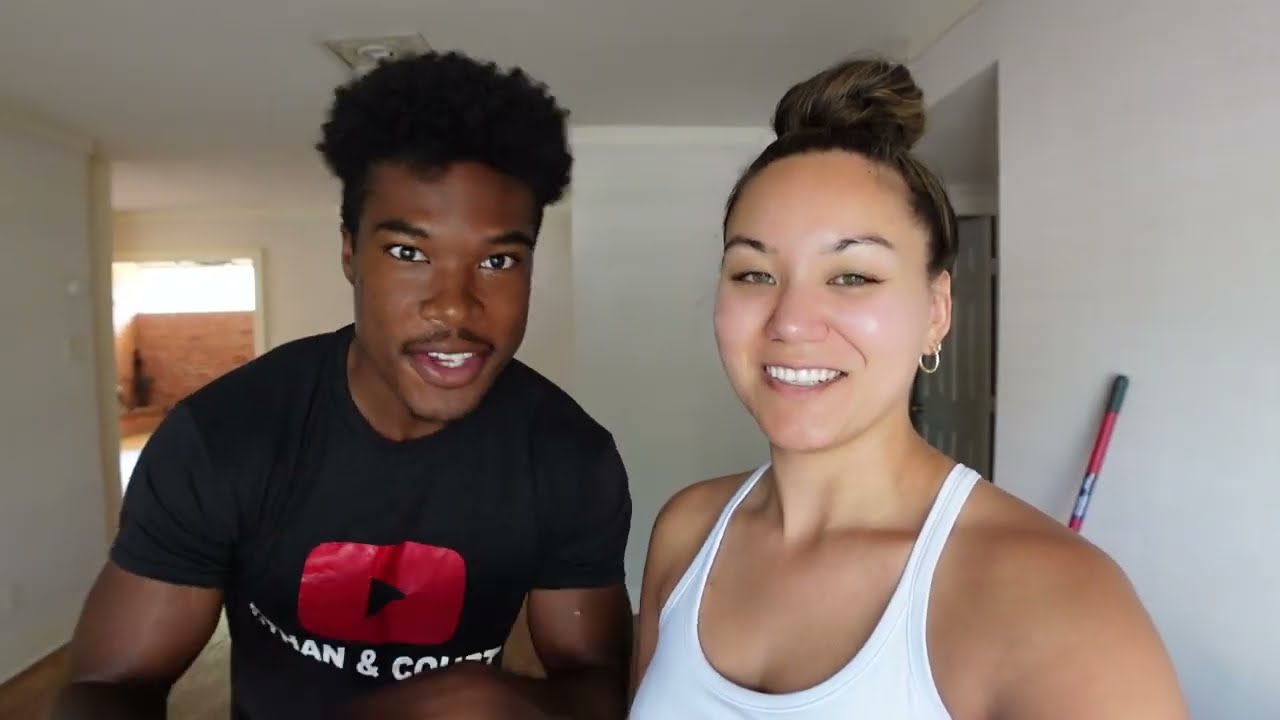In this detailed photograph, we see two young, athletic individuals who appear to be in their 20s, amicably looking at the camera in what seems to be a living area, possibly an apartment. The person on the left is a young African American man with medium dark skin, sporting a slightly mid-length Afro hairstyle that is cropped close on the sides but higher on the top. He has a slight smile and an open-mouthed, relaxed expression, wearing a black t-shirt featuring a red rectangle with a black triangle symbol—reminiscent of a YouTube play icon—and white writing underneath, though the text is not legible. He appears muscular and the image captures him from head to mid-torso.

Next to him on the right is an attractive young woman of mixed ethnicity, likely Latino, with slightly lighter skin. Her dark hair is neatly pulled back into a top knot, showcasing her nicely arched dark eyebrows. She smiles warmly at the camera, conveying a sense of ease and happiness. She is adorned with gold hoop earrings and is dressed in a white tank top that highlights her fit and toned physique. The photo similarly frames her from the head to upper torso.

The background reveals an off-white interior with a doorway behind the young man, through which a red wall with white accents is visible, possibly indicating another room or an outdoor space. Additionally, there is an object leaning against the wall that resembles the top of a hockey stick or some kind of handle.